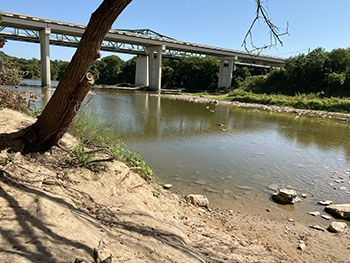This photograph captures a scene from a dirt bank beside a very shallow, slim river, clear enough to reveal a rock bed through the water. The river, which has a dark greenish-brown tint, flows gently, bordered by scattered rocks and leaning trees on both sides. A particularly notable tree trunk extends into the upper left-hand corner, seemingly reaching towards the viewer. The foreground presents a rugged, dirt-filled hill, gradually transitioning to a more verdant backdrop where grass and numerous trees flourish. Dominating the middle ground is a large, concrete bridge with elevated roadways, standing out with its tan and brown hues. The entire scene is bathed in sunlight under a clear, blue sky, emphasizing the serene yet rugged nature of the landscape.